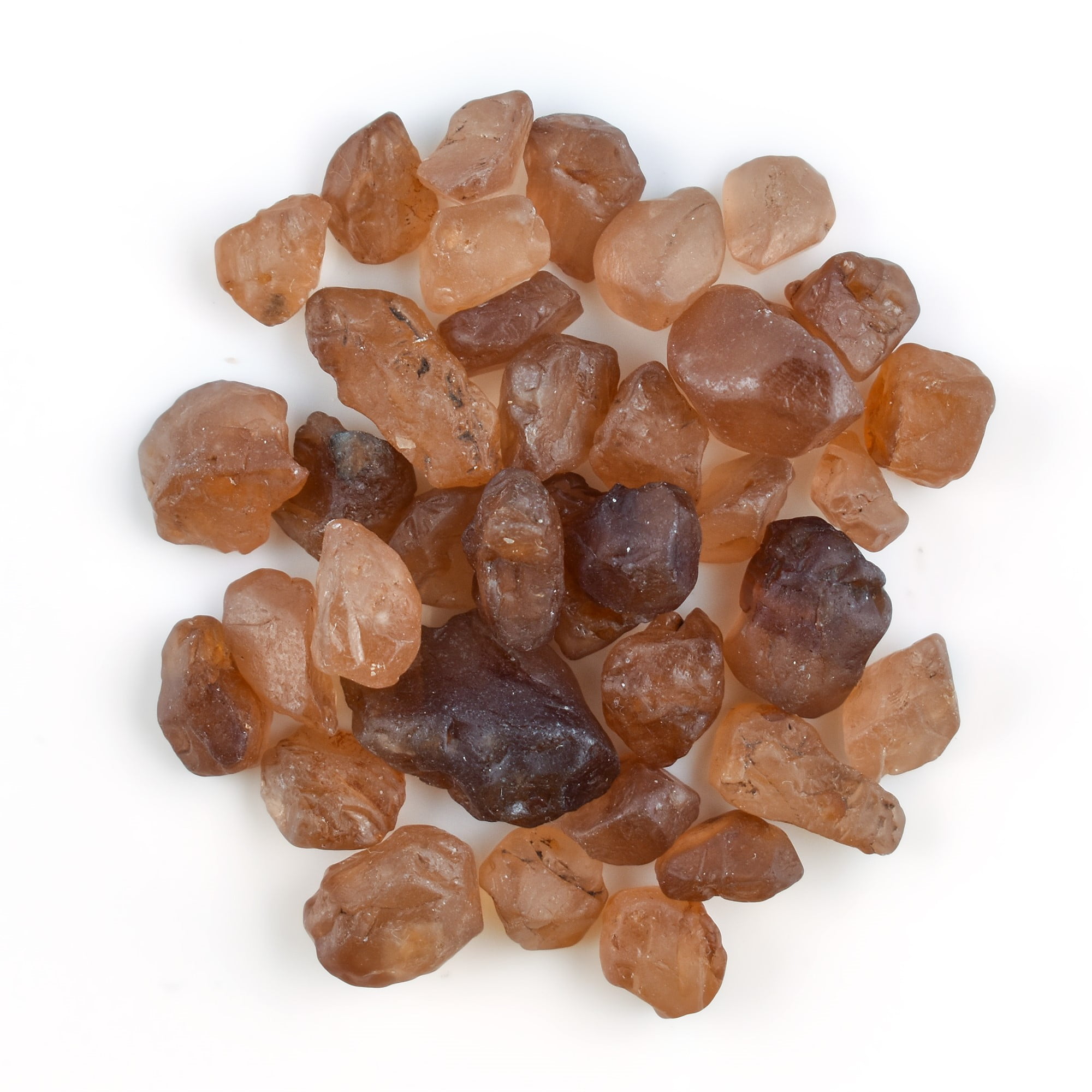This image features a collection of small, pebble-sized rocks or gemstones scattered uniformly on a white background. Ranging in shades from tans and light browns to rich golden browns and almost black, darker browns, these stones exhibit a semi-translucent, crystal-like appearance, though they are opaque. The rocks are variously shaped—some are square-ish, cylindrical, or rounded—while the darker ones, predominantly in the center, contrast with the lighter hues around them. Despite their rough, natural state, they appear slightly glossy, possibly from wind or water erosion. Approximately 30 to 40 stones are depicted, tightly clustered together, with their organic, somewhat amorphous forms reflecting light subtly, contributing to the overall aesthetic of the photo.